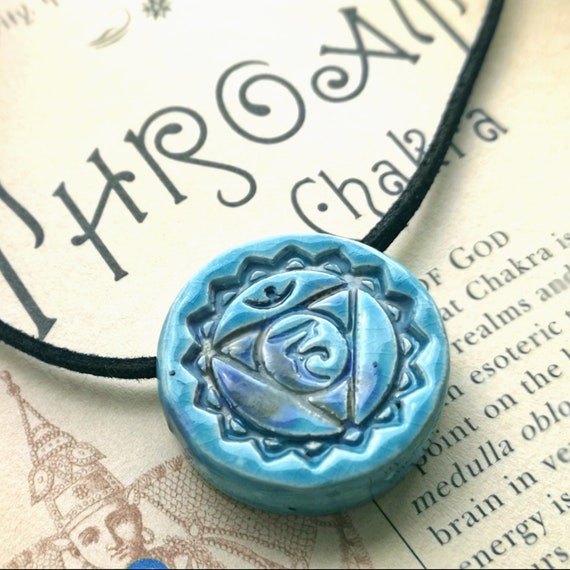The image is a color photograph in portrait orientation, closely capturing a pendant necklace centered near the bottom of the frame. The pendant is a handmade round ceramic disc, light turquoise in color with an aqua-blue iridescent glaze, giving it tones of blue and gold. It features a radiant sun design with "teeth" around the edge, symbolizing the sun. Inside the sun, an engraved inverted triangle is present, encasing a smaller circle with intricate characters, possibly in another language or representing symbolic elements, resembling an upside-down saber sword.

The pendant is threaded with a black leather strap, entering from the left, looping through the top of the pendant, and exiting in a curve towards the top right. This strap extends as a thin rope on both sides. The pendant rests on a light brown, parchment-like page that appears new and clean. In the left-hand corner of the page, there is an illustration of a wizard or Hindu goddess, wearing a pointed hat. The upper portion of the page contains text, with visible words including "chakra" and potentially other terms that hint at the pendant’s spiritual or symbolic significance. The style is a realistic and representational form of product photography, emphasizing the pendant’s intricate design and the textual and illustrative details of the background.